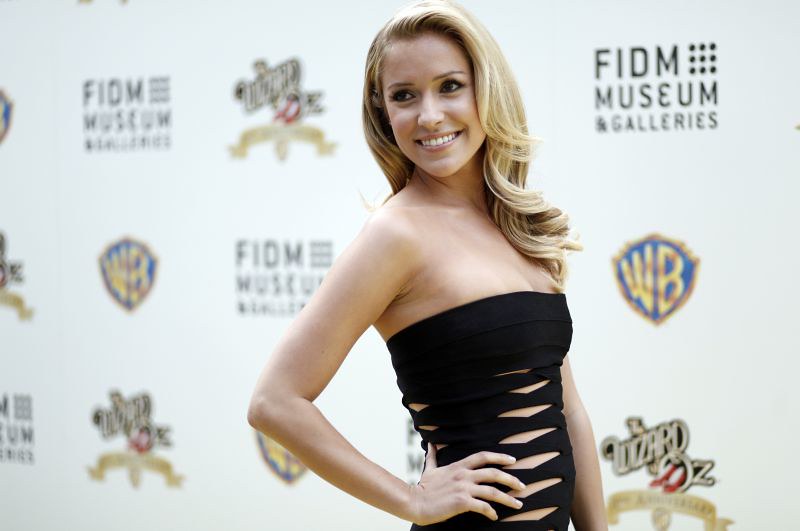In this image, a young, thin Caucasian woman with long, wavy blond hair is posing in front of a white backdrop adorned with repeated logos, including those of Warner Brothers, the Wizard of Oz, and FIDM Museum and Galleries. She is dressed in a strapless, shoulderless black dress that features stylish cutouts along the front, sides, and back, revealing a hint of skin beneath. Her left hand is confidently positioned on her hip, while her right arm hangs loosely by her side. With her head slightly tilted back, she gazes off to the side, smiling. The image appears to be taken at an event or award show.